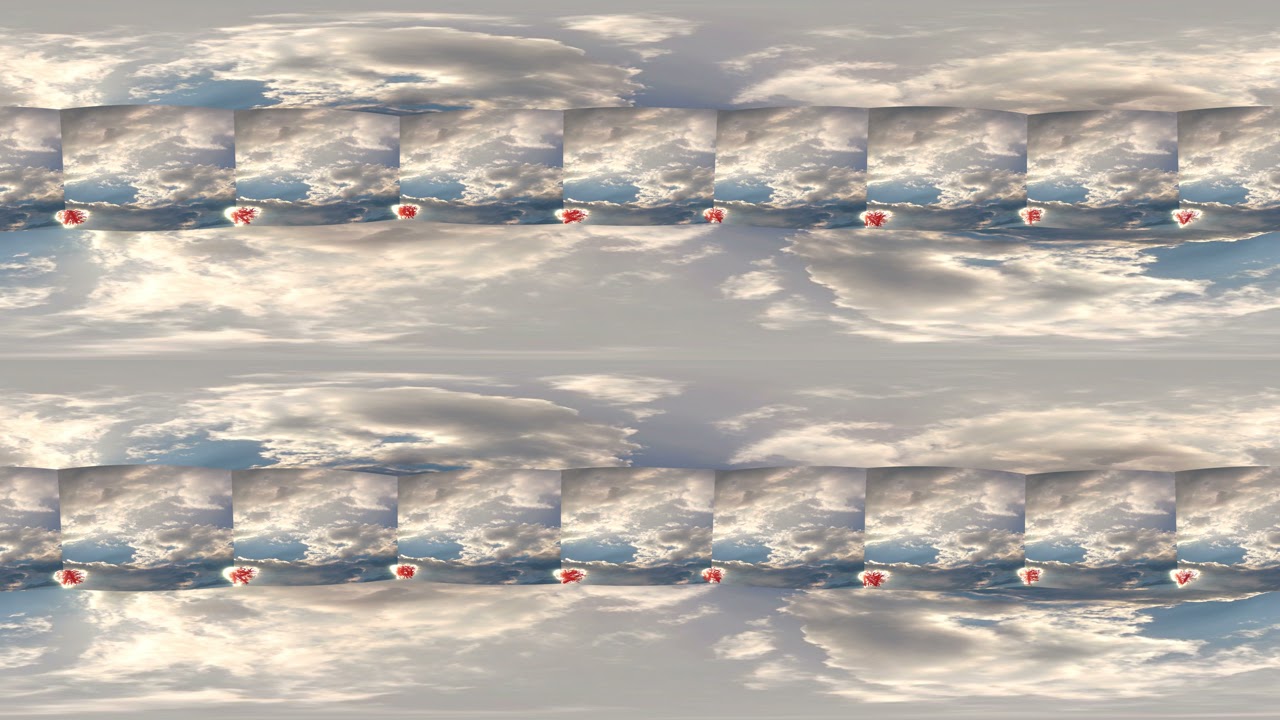The image is a digitally manipulated artwork featuring a sky scene and repeated cloud formations. Two identical horizontal strips are stacked vertically against a backdrop reminiscent of what one might view from an airplane at 30,000 feet, showcasing a gray, milky sky filled with puffy cumulus and cirrus clouds. Each strip contains nine small, framed cloud images evenly spaced across the width of the piece, intersected by tiny red stars that appear to be drawn with a marker. These stars are positioned between each frame, suggesting a purposeful selection by the artist. The repetitive, layered arrangement combined with these artistic markings creates a symmetrical and surreal visual effect, possibly highlighting the interplay between natural elements and digital artistry.